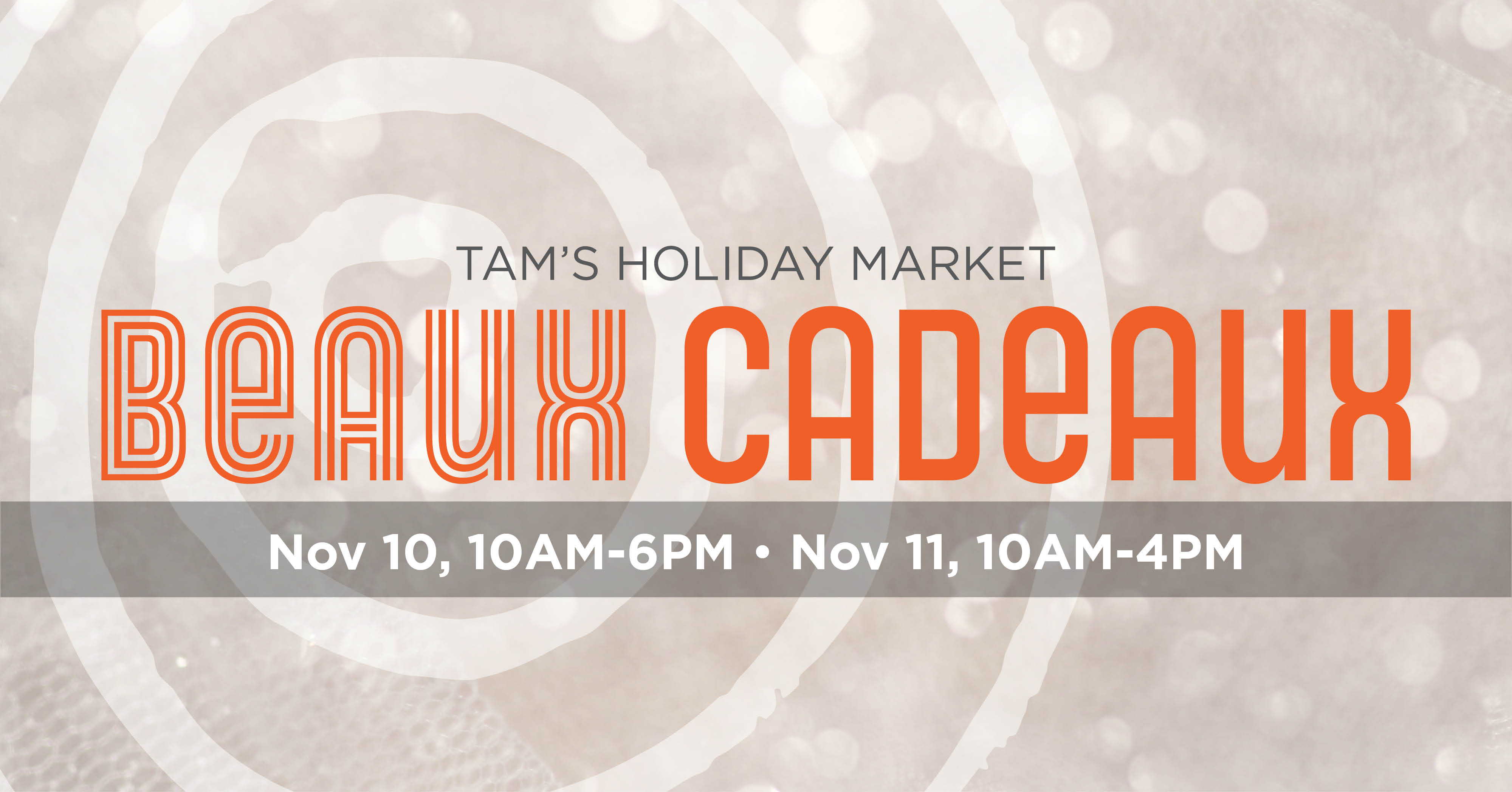This image is an advertisement for "Tams Holiday Market," prominently displayed in small, darker gray text at the top center of the visual. Below this title, the phrase "Beaux Cadeaux" is strikingly featured; the word "Beaux" is designed with outlined orange letters, while "Cadeaux" is written in solid orange letters. These words are aligned, with "Beaux" on the left and "Cadeaux" on the right. Beneath "Beaux Cadeaux" is a semi-transparent gray banner stretching horizontally across the image, with white text indicating the event dates and times: "November 10, 10 a.m. to 6 p.m." and "November 11, 10 a.m. to 4 p.m." The background is primarily beige, adorned with white dots scattered throughout. On the left side of the background, there's a series of white concentric circles, reminiscent of a bullseye pattern, adding a decorative element to the overall design.